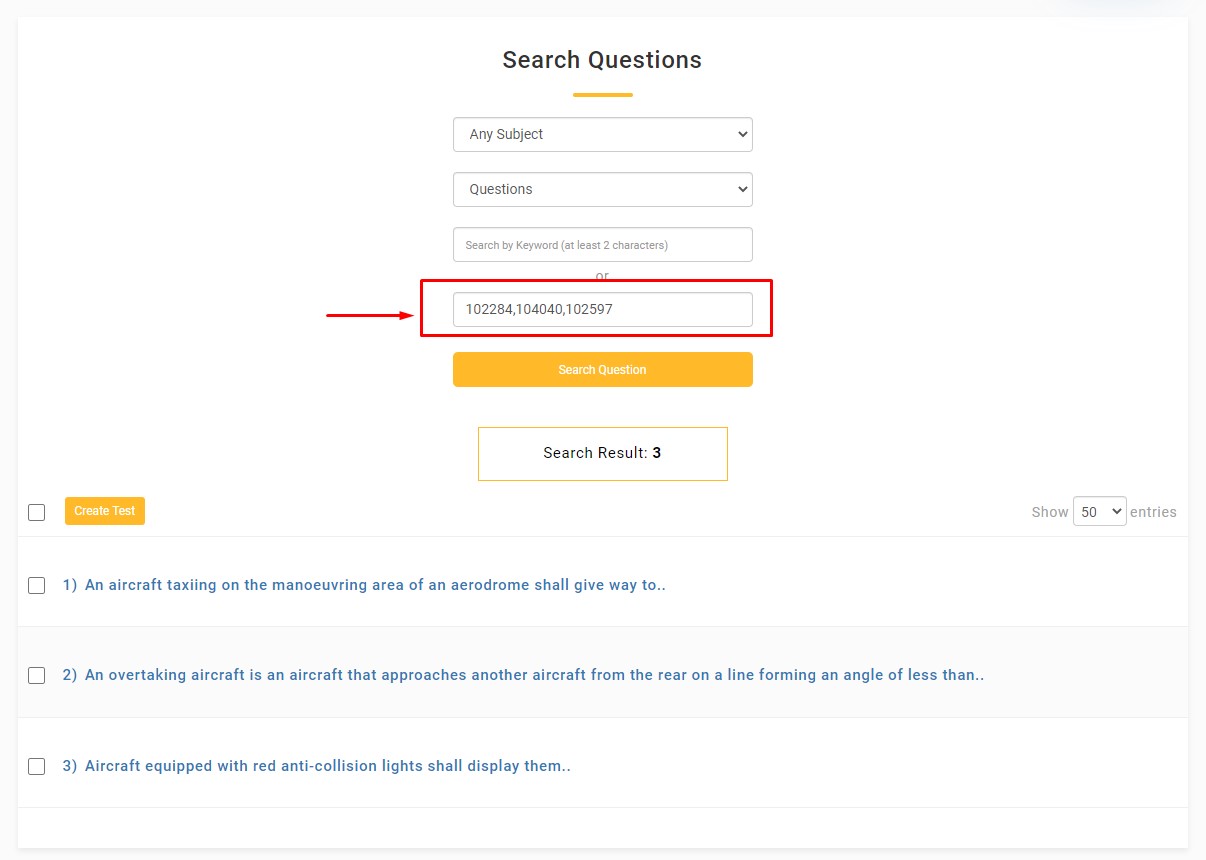This image captures a screenshot of a website functioning as a search question database. The layout includes four distinct search boxes, each serving a unique purpose. 

1. The first box offers a comprehensive search option for any subject matter.
2. The second box is labeled "Questions," dedicated exclusively to querying specific questions.
3. The third box provides an input field for keywords, where users must type at least two characters to initiate a search.
4. The fourth and final box displays a sequence of numbers—102284, 104040, and 102597—though it lacks any explanatory context for their significance. This particular box is prominently highlighted in a red rectangle and features an arrow pointing towards it.

Beneath the boxes, there is an interactive button labeled "Search for Questions."

The image reveals that a search was conducted, yielding three results. Each search result appears to relate to aviation:

1. "An aircraft taxiing on the maneuvering area of an aerodrome shall give way to..."
2. "An overtaking aircraft is defined as an aircraft that approaches another from the rear on a line forming an angle of less than..."
3. "Aircraft equipped with red anti-collision lights shall display them..."

The highlighted numbers and their associated search results imply there could be a connection or reference to aviation regulatory standards or identification codes.